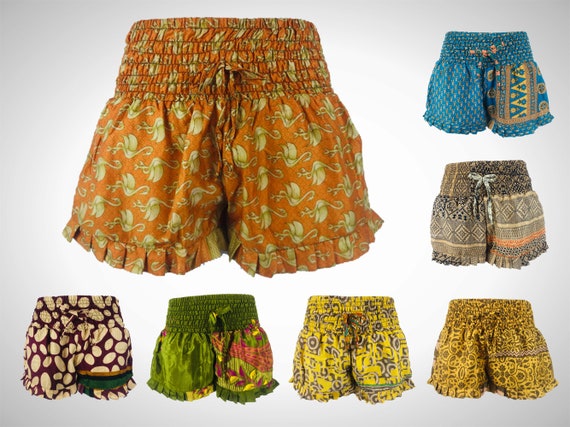The photograph displays a collection of seven pairs of fabric shorts with a distinct vintage look, evoking the style of old-school bloomers. Each pair features a cinched waist with a tie and ruffled thigh openings, giving them a shabby chic aesthetic. The largest pair, prominently positioned on the top left, is orange with a seersucker-like texture, adorned with swirling light-colored designs, and includes a tie for waist adjustment. To its right, a blue pair stands out with a complementary yellow background design.

Below the blue pair, a set of beige, tan, and salmon-striped shorts with a light-colored sash can be seen. Adjacent to these, a tan pair of shorts presents an intricate, yet indistinct, pattern. Directly below the orange shorts, another pair appears in yellow, embellished with dark green decorative designs.

To the left, there's a pair featuring an asymmetrical design: one leg and the waist are dark green, while the other leg is a mix of light green, dark green, and red or coral. The final pair in the bottom left corner has a dark brown background with a delicate pattern of light tan leaves, giving the appearance of falling motions.

These shorts, while diverse in color and pattern, share the same gathered waist and ruffled thigh details, creating a cohesive and charmingly antiquated look.